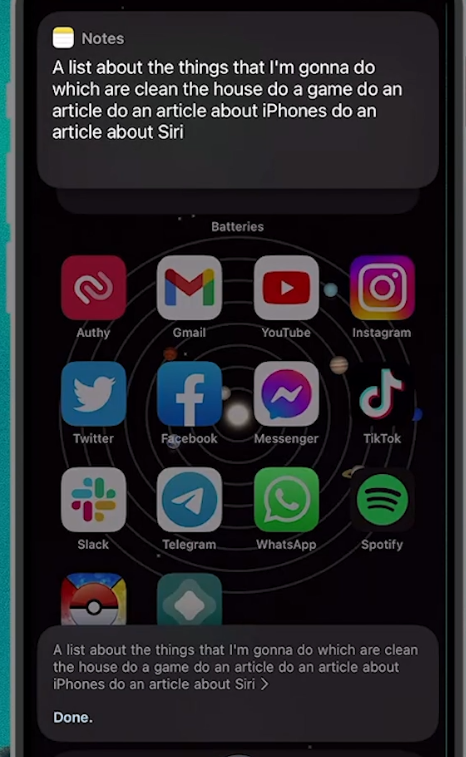This image is a screenshot taken from a cell phone. At the top of the screen, an open note is visible, which contains a list of tasks. The note reads: "A list about things that I'm going to do: clean the house, do a game, do an article, do an article about iPhones, do an article about Siri." The background of the screenshot shows various application icons, including TikTok, Facebook, Twitter, Facebook Messenger, WhatsApp, Spotify, Telegram, Pokemon Go, Gmail, and YouTube. At the very bottom of the image, a gray message bubble displays the same text from the note: "A list about the things I'm going to do: clean the house, do a game, do an article, do an article about iPhones, do an article about Siri." In the bottom left-hand corner, the word "Done." appears.